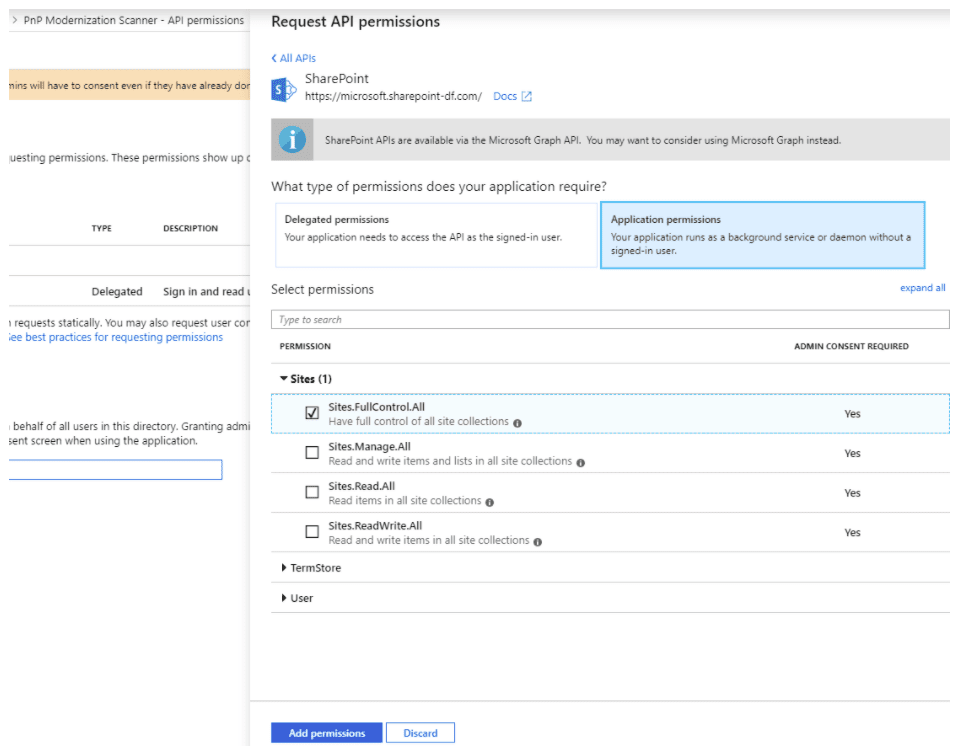### Detailed Caption for the Image

The image displays the "API Permissions" page of a web interface. 

- **Top Section:**
  - The header reads "API Permissions – API Permissions."
  - On the right is a button labelled "Request API Permissions."

- **Left and Middle Section:**
  - A blue left-pointing arrow labelled "All APIs."
  - Beneath this, it reads "PMP Moderation."
  - A yellow box containing partially cut-off text follows, mentioning something about consent requirements that are not fully visible.
  - More cut-off text is visible further down.

- **Body Section:**
  - Below the "All APIs" text is "SharePoint Microsoft SharePoint df.com docs."
  - A small blue box with an 'S' inside is adjacent to a blue circle containing an 'i'.
  - A grey box next to these icons states: "SharePoint APIs are available via the Microsoft Graph API. You may want to consider using Microsoft Graph instead."

- **Permission Selection Section:**
  - The text "What type of permissions does your application require?" followed by options to select "Delegated Permissions" or "Application Permissions." The "Application Permissions" option is currently selected and highlighted in blue.
  - The text "Select Permissions" appears with an accompanying search box with the placeholder "Type to search."
  - A table follows with columns labelled "Permission" and "Admin Consent Required," including a dropdown menu showing "Sites 1" with several selectable checkboxes. Each checkbox has "yes" next to it, indicating admin consent.
  - Further dropdown boxes labeled "Term Store" and "User" are listed beneath, but they are not expanded.

This image depicts the detailed user interface elements related to setting API permissions, offering a range of configuration options within a structured layout.